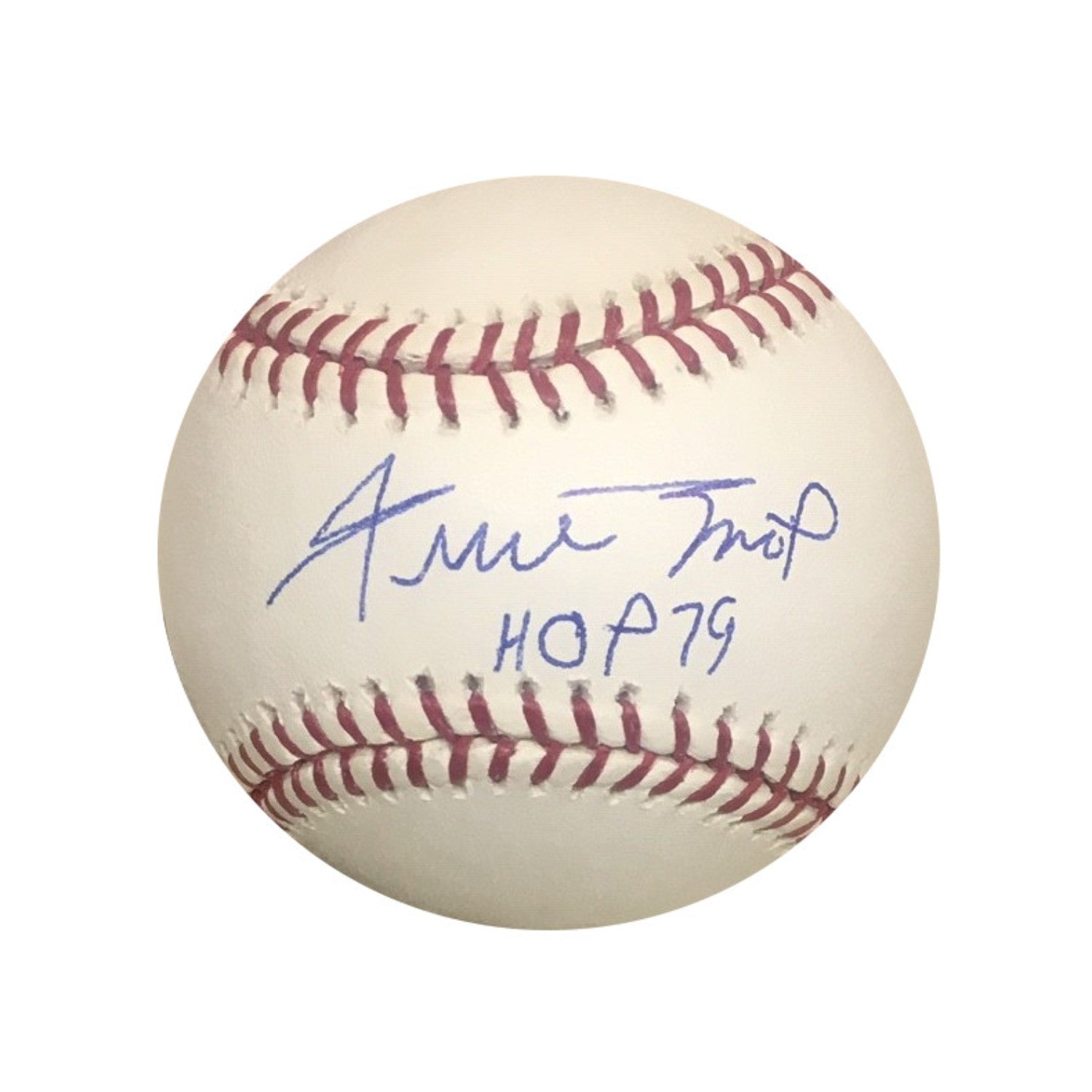The image features a classic baseball positioned against a completely white, featureless background. The baseball appears aged, displaying a dull, off-white color with faded maroon lacing arranged horizontally from left to right. Prominently in the center of the ball is a difficult-to-read signature that loosely resembles either "IAMITTMO" or "AMORENTROP," followed by the annotation "HOP 79." Despite its vintage appearance, the baseball shows no signs of wear or tear, maintaining its traditional aesthetic with well-defined stitching visible at the top and bottom.